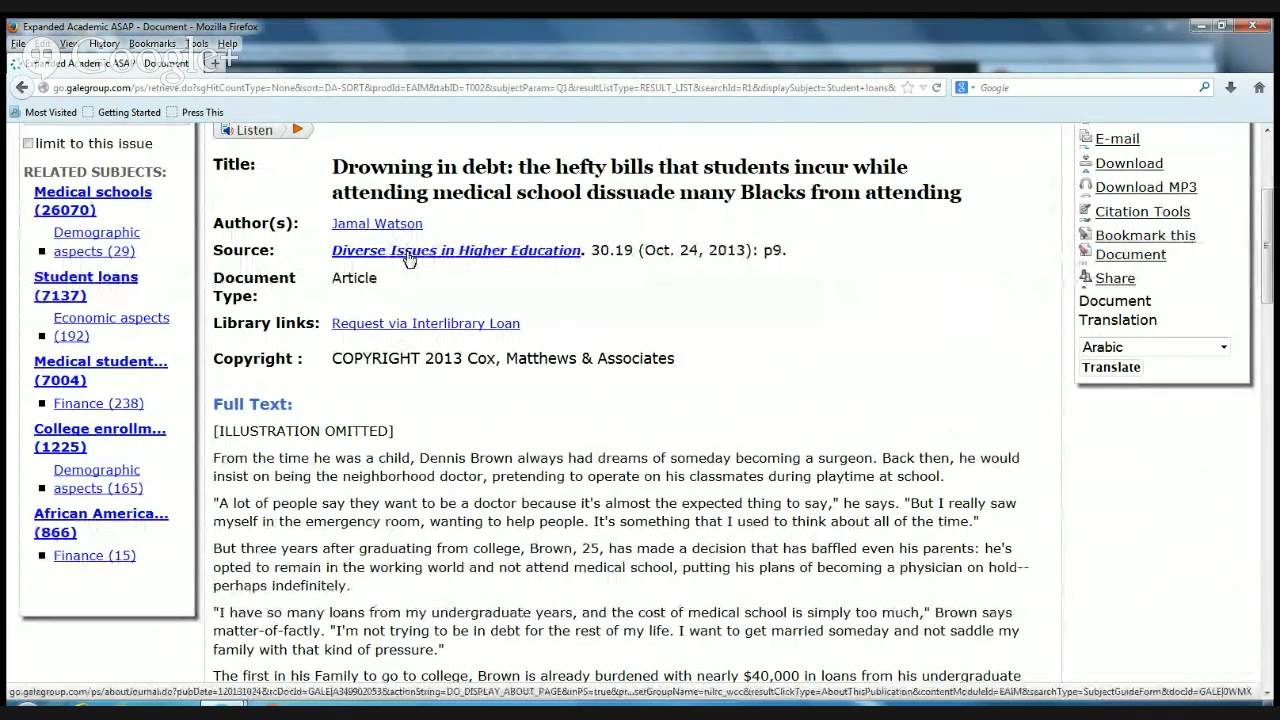This is a screenshot of a Firefox browser window opened to the website galegroup.com. The user appears to be reading an expanded academic ASAP document. The article's title is "Drowning in Debt: The Hefty Bills that Students Incur While Attending Medical School Dissuade Many Blacks from Attending," authored by Jamal Watson. The mouse cursor is hovered over the source, which is "Diverse Issues in Higher Education." The document is classified as an article and offers a library link for requesting the text via interlibrary loan. It is copyrighted in 2013 by Cox, Matthew, and Associates. The beginning of the article's text is visible, indicating that illustrations have been omitted. On the left side of the screen, a dropdown menu lists related subjects including medical schools, student loans, medical students, college enrollment, and African-Americans. On the right side, various options are available such as emailing, downloading (both as text and MP3), citing, bookmarking, sharing, and translating the document.